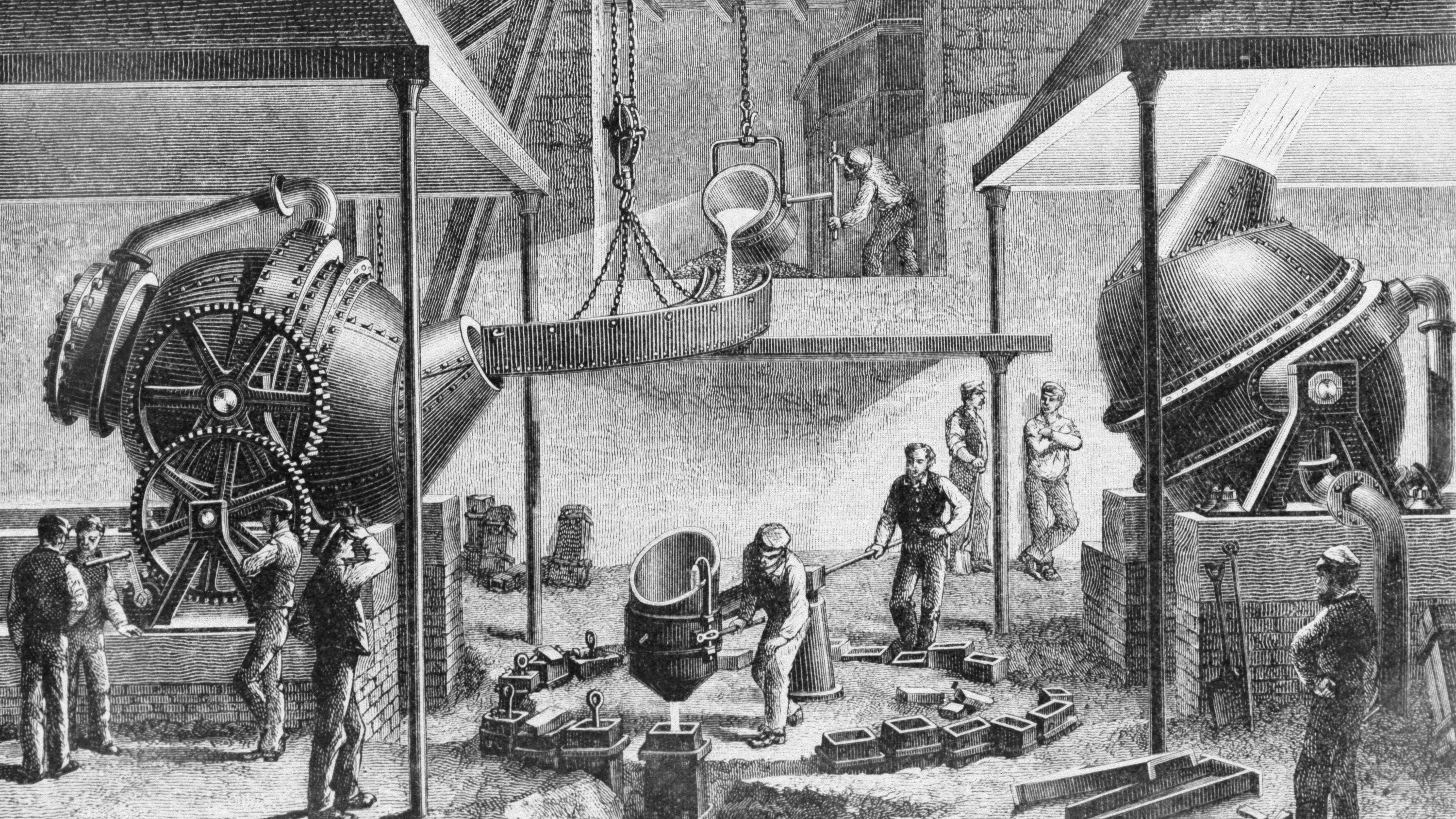The image is a black-and-white old-fashioned illustration depicting an active smelting facility. The scene is detailed, set in a horizontal landscape orientation. Central to the image, there is a large funnel suspended from chains, into which a worker on the top middle platform is pouring a white, molten substance from a bucket. This funnel is connected to a series of large, gear-operated machines on the left and right, which have conical ends that are emitting steam or fire.

The left side features a significant machine with large, visible gears and a barrel-like structure. Below it are brick walls supporting the machinery. To its right, a group of four workers is seen engaged in conversation, with one of them looking up towards the machinery.

In the center of the image, towards the bottom, another worker is seen pouring molten material from a large cylinder into a series of block forms on the ground. These forms are surrounded by stakes and metal pieces. Behind this central worker, another man operates a crank wheel that controls the flow of the molten substance from the funnel above.

To the far right, another large machine with a conical end and emitting steam or fire is supported by brick walls. Several workers are present here as well, including one standing with a shovel, overseeing the operations. Throughout the illustration, gears, pulleys, and various mechanical components emphasize the industrial nature of the setting.

Overall, the illustration captures the meticulous and labor-intensive atmosphere of a historical smelting facility, with detailed emphasis on the machinery and the workers' coordinated efforts.